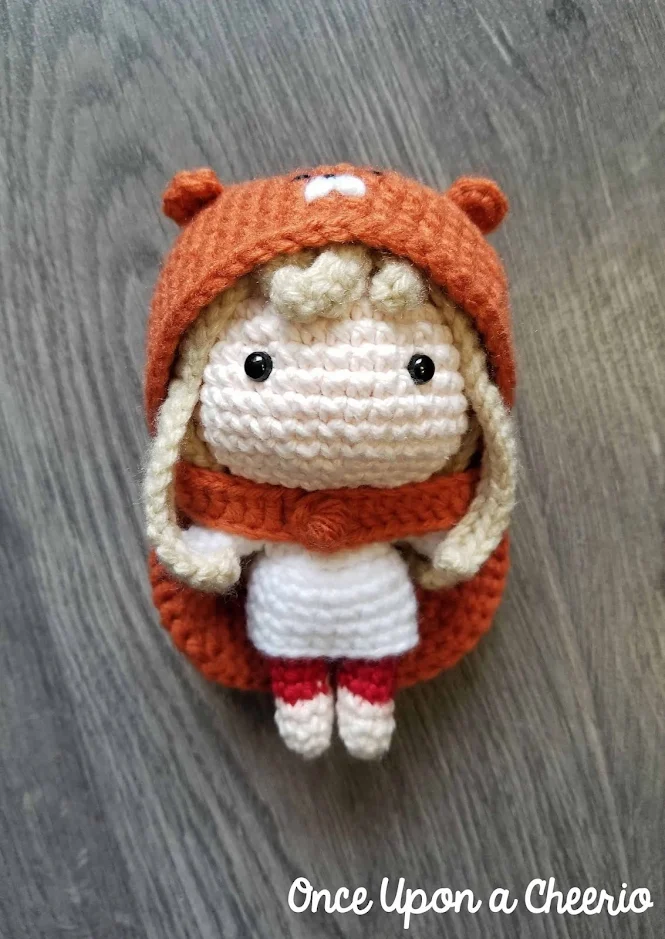The image features a small, intricately crocheted doll resembling Little Red Riding Hood, prominently occupying around two-thirds of the frame. This soft toy, viewed from a top-down perspective, is placed on a table, which may be wooden or faux wooden. The doll has a cream-colored, slightly crude yet charming design, characterized by black button eyes without any other facial features. She sports long blonde hair, styled in braids, and wears a white dress paired with red and white leggings and shoes. Over her dress, she dons a red cloak with an integrated hood that mimics a bear's head, complete with ears and a white snout. The text "Once Upon a Cheerio" is displayed in white cursive lettering at the bottom right corner of the image, adding a finishing touch to this cozy, handmade scene.